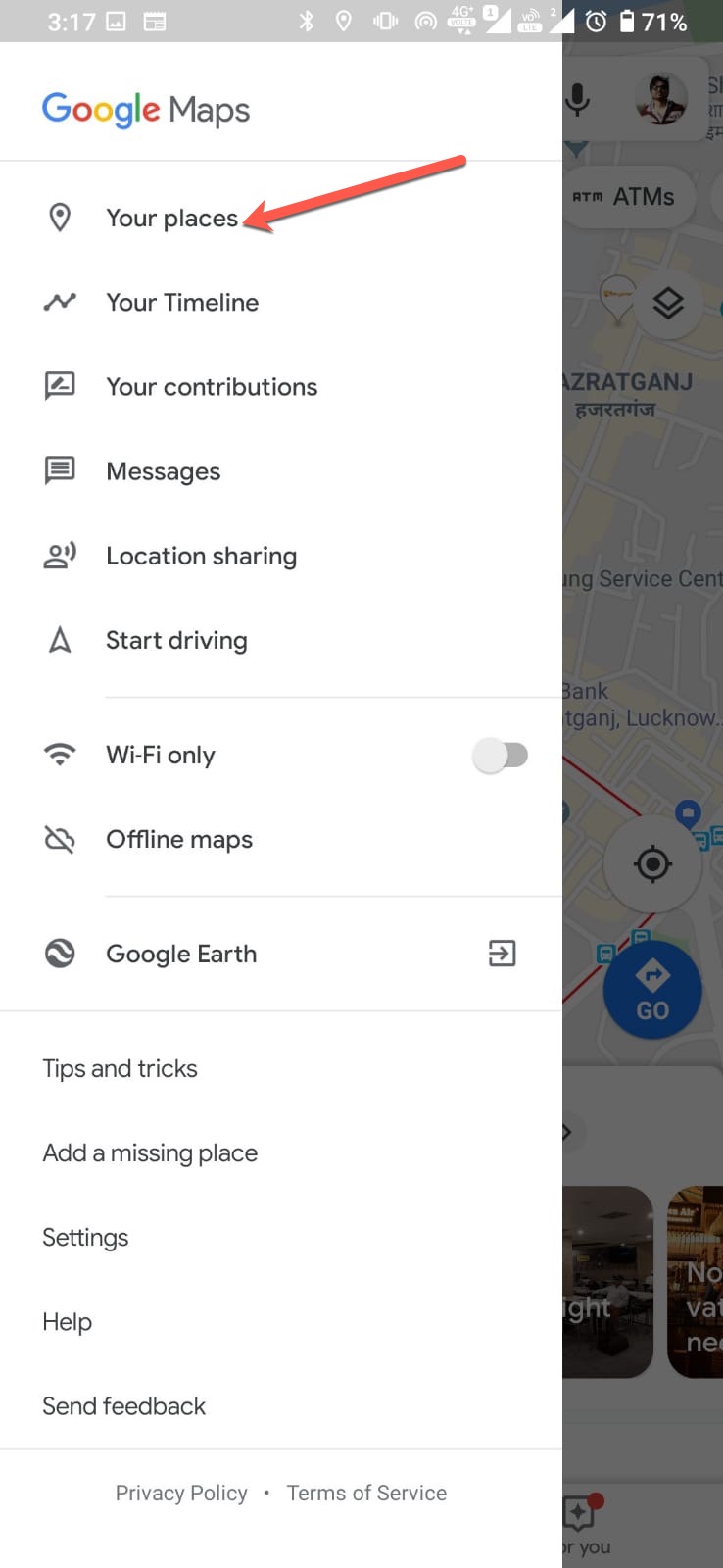This image is a screenshot of a smartphone displaying the Google Maps application. The device has a battery level of 71% along with several other small, indistinguishable icons at the top right corner of the screen. At the top of the app, the title "Google Maps" is displayed. Beneath the title is a horizontal bar, below which the text "Your Places" is highlighted by a long, slim red arrow pointing towards it.

Following this, a list of options is visible, each with a representative icon to its left. The list includes:

- "Your Timeline"
- "Your Contributions"
- "Messages"
- "Location Sharing"
- "Start Driving"
- "Wi-Fi Only," which features a gray toggle switch set to the left. 
- "Offline Maps"
- "Google Earth"
- "Tips and Tricks"
- "Add a Missing Place"
- "Settings"
- "Help"
- "Send Feedback"

At the bottom of the screen, text links for "Privacy Policy" and "Terms of Service" are visible, completing the menu options.